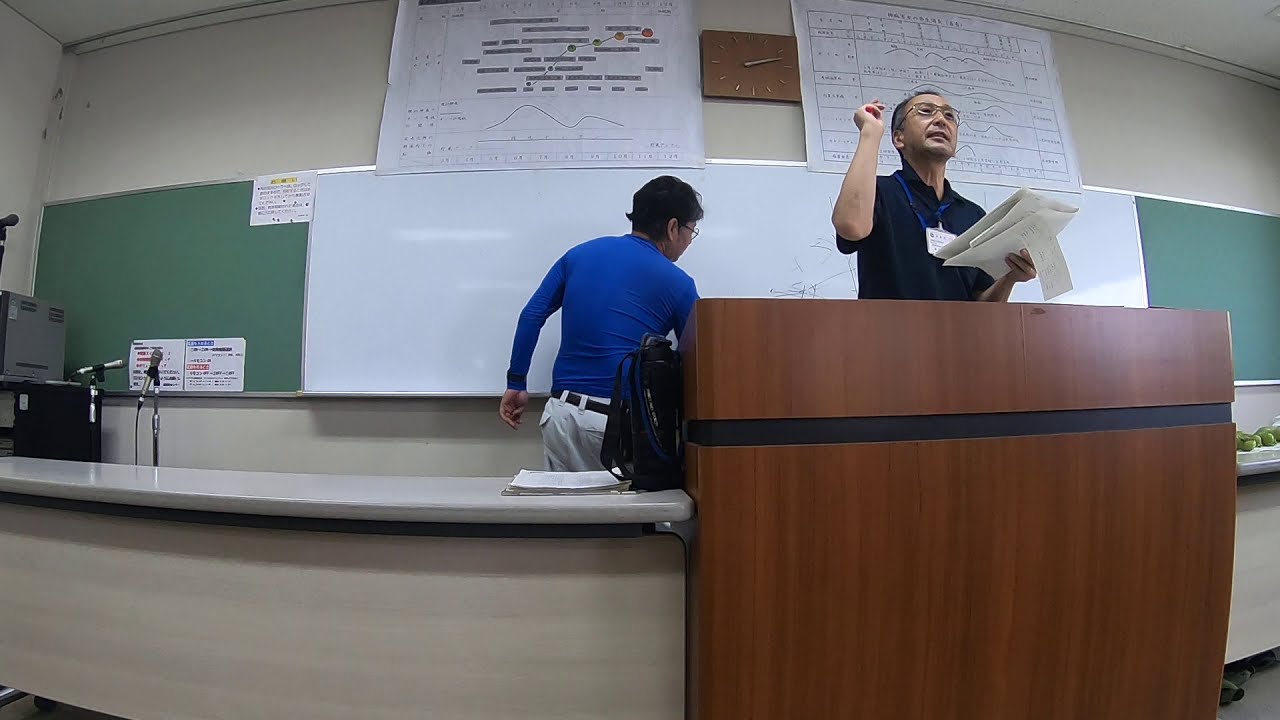This landscape photograph captures a professional, classroom-like setting. On the right side of the image, an older Asian man, dressed in a blue collared shirt with a lanyard around his neck and wearing glasses, stands at a brown wooden lectern. He is holding papers in his left hand and has his right hand raised, possibly making a point during a lecture or meeting. Behind him, the board is divided into three sections: the left and right sections are green chalkboards, while the central section is a whiteboard intended for marker use. 

A second man, wearing a long-sleeved blue shirt and white pants, faces the whiteboard with his back to the camera as he writes on it. Above the board, a brown clock is centered, flanked by large posters or charts with graphs on either side. To the far left, a beige table holds a black briefcase, and microphones along with hardware are visible. Several white signs with black, red, and yellow text are taped to the green chalkboard, although the contents of these signs are not legible.